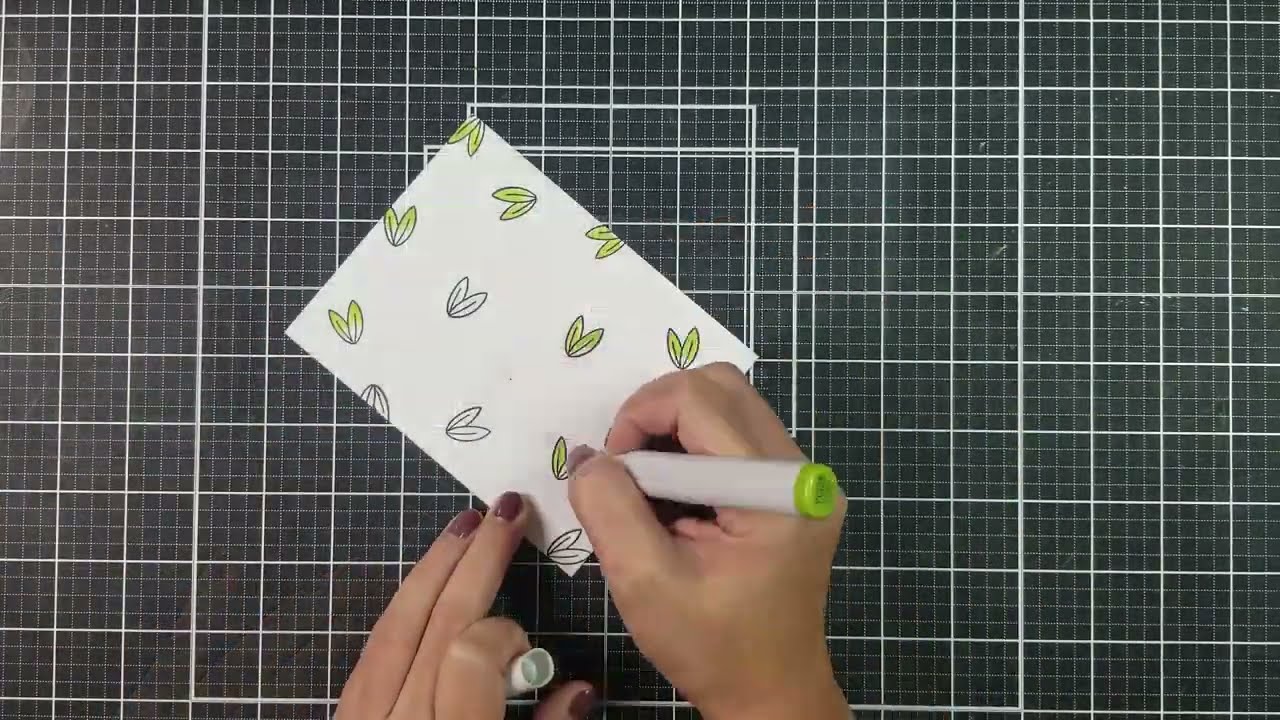In this horizontal rectangular image, a woman with dark red to magenta fingernail polish is depicted using a white marker with a green tip to color in a small, square piece of paper. The paper features a repeating pattern of leaves, some of which have already been shaded in yellow, green, and white. Her right hand holds the marker while her left hand clutches the cap. The background displays a meticulous grid pattern of white and black squares, each subdivided into smaller squares that form a secondary grid, adding a detailed and intricate backdrop to the scene. You can see only her wrists and hands, focused intently on her precise coloring work.